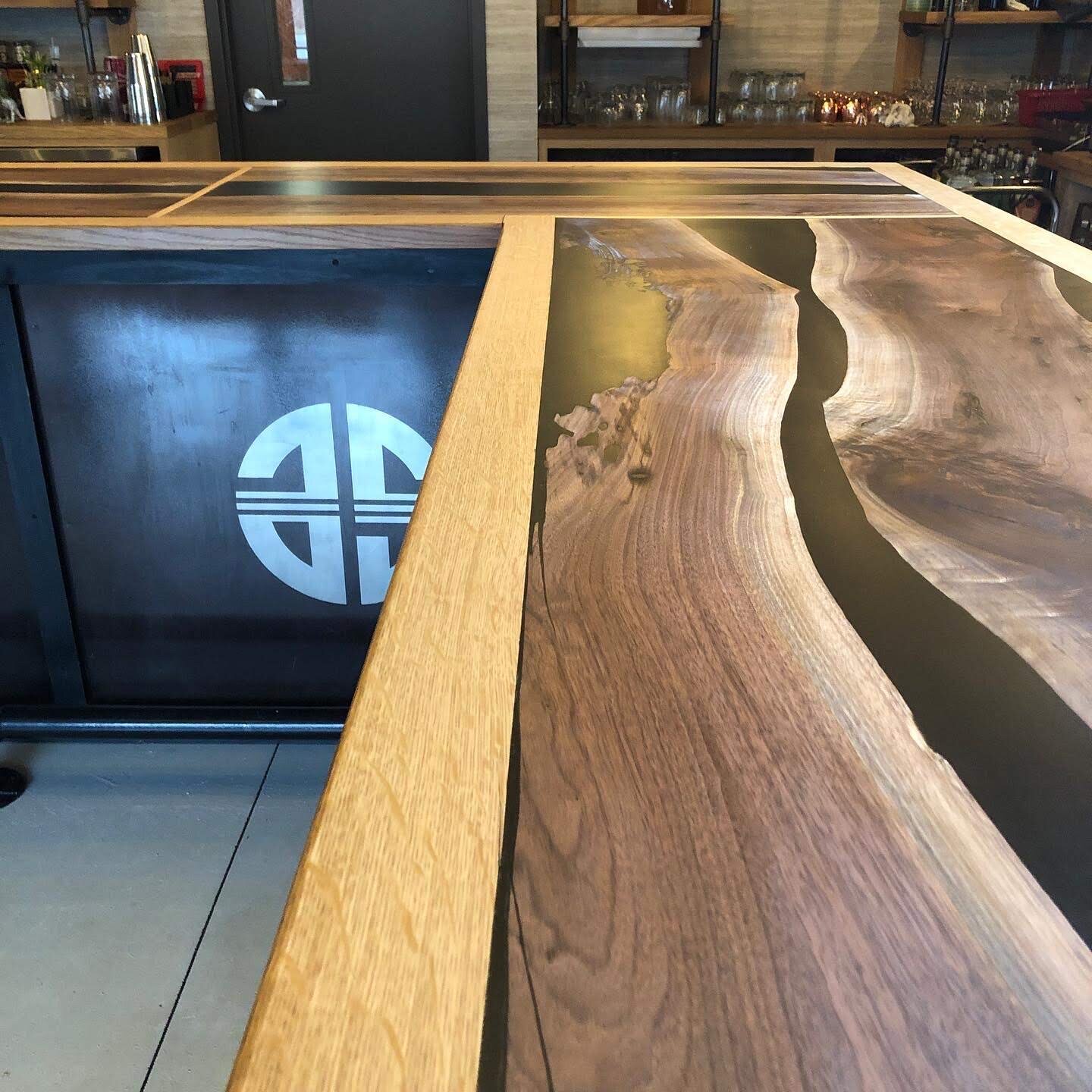The photograph captures a bar's L-shaped tabletop, extending from the bottom of the frame and turning off to the left. The countertop is comprised of light brown wood panels featuring distinctive black marbling, giving it a unique and somewhat unconventional appearance. The bar's side panel is black, showcasing a partially obscured circular logo that seems to read "GS." In the background, several tables or stations are visible, adorned with glassware and stainless steel mixing cups, as well as a container of salt. There's a closed, off-black door with a vertical rectangular window and a silver knob. Notably, the bar countertop itself is clear, devoid of any napkins, cups, or patrons, emphasizing a clean and orderly atmosphere.